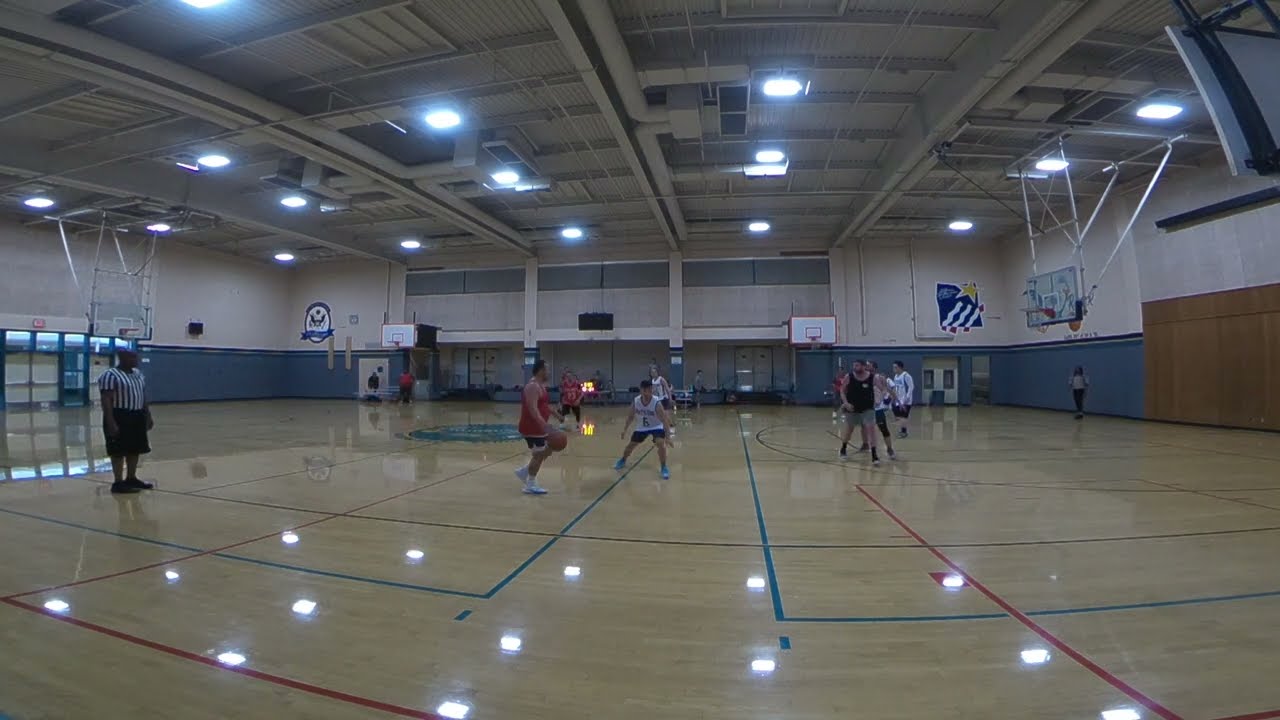The photograph depicts a vibrant, brightly lit gymnasium during an informal basketball game, possibly at a YMCA or a community rec center. The large indoor space features a polished wood floor marked with blue and red lines, reflecting the ceiling lights. Prominent in the image are two main basketball hoops mounted on what appear to be sliding tracks, with two smaller hoops fixed against the distant wall. The game's six players are dressed in various non-uniform outfits, typical of a casual pick-up game. A man in blue shorts and a red tank top is dribbling the ball, closely defended by a player in blue shorts and a white tank top. Two referees are present: one positioned near the middle-left of the court and another referee visible farther in the background. The gym's walls are painted blue on the bottom half and white on the top, resembling a large warehouse with a high ceiling. Natural daylight streams in from the left side, adding to the well-lit atmosphere of the venue.